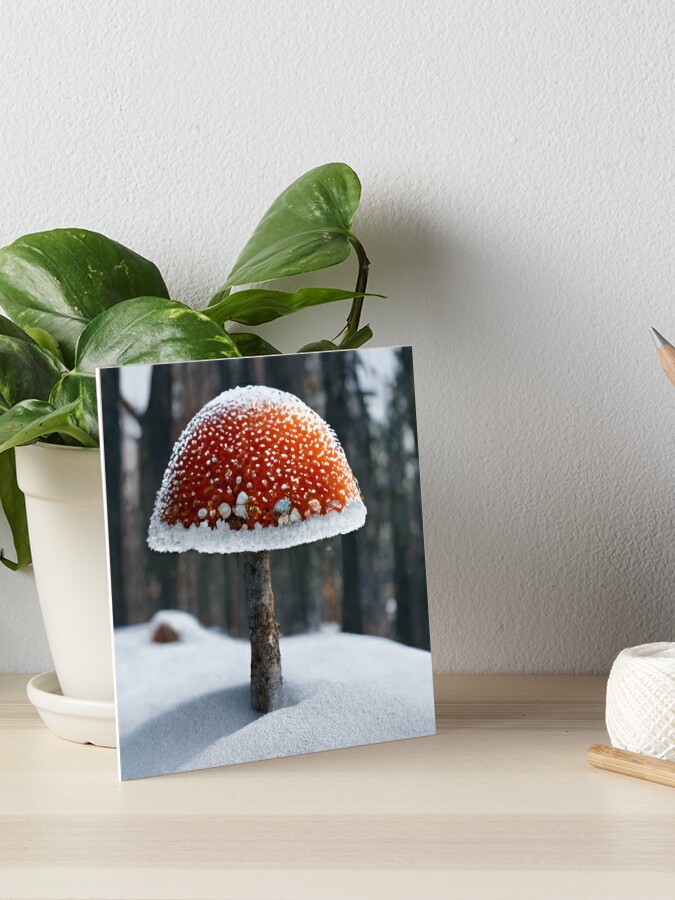The photograph captures a detailed desk scene, where the focal point is a small picture of a red mushroom with a brown stem, propped up against a beige potted plant with large, waxy green leaves. The mushroom, prominently displayed in the picture, is covered in a delicate frost, giving its cap an icy, snow-covered appearance, with snow collecting at its base. Behind the icy mushroom image, a wintery forest is faintly visible, bare of leaves, adding to the chilly atmosphere. The potted plant, partially obscured by the picture, provides a lush green contrast, enhancing the overall composition. The scene appears to be set on a desk up against a wall, creating a cozy yet picturesque vignette.